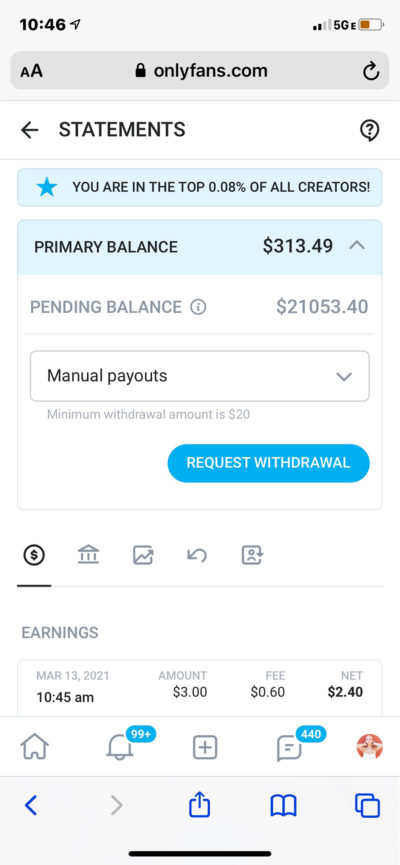The image depicts a screenshot from a smartphone, likely taken from an OnlyFans.com account. In the top right corner, the battery icon indicates it is at 50% charge, and the current time is 10:46 AM. The screenshot shows the 'Statements' page, implying details of owed payments to a performer. At the top, a blue star highlights the user's rank, stating, "You're in the top 0.08% of all creators."

Below this, the "Primary Balance" is prominently displayed in bold, all-capital letters with a blue background, showing an amount of $313.49. Adjacent to this is the "Pending Balance," shown in grey, amounting to $21,053.40. A drop-down box for payout options follows, currently set to "Manual Payouts," with a note that the minimum withdrawal amount is $20. Following this section is a blue button labeled "Request Withdrawal."

The page is currently on the "Earnings" tab, suggested by the all-capitalized, greyed-out "EARNINGS" label. Below, a transaction is detailed: on March 13, 2021, at 10:45 AM, an earning of $3 was recorded, with a fee of $0.60, netting $3.40. 

Icons arrayed at the bottom of the screen include 'Home,' 'Alerts' (showing 99+ notifications), a 'Plus' sign within a square, a comment icon displaying 440 replies, a back arrow, a share button, a bookmark option, and a button for multiple tabs.